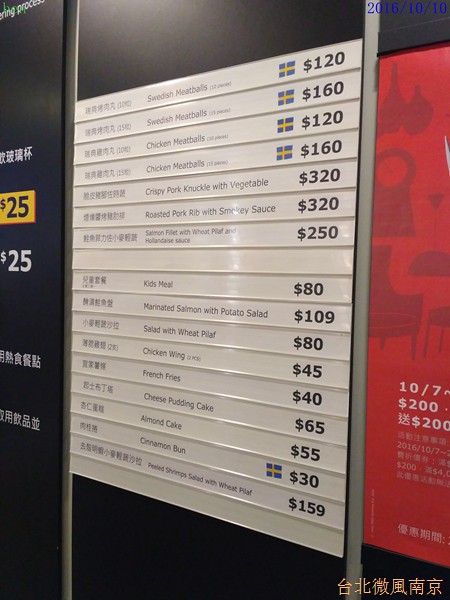The photograph is a colorful and detailed image with a watermark at the bottom made up of six Chinese characters. The focal point of the image is a prominent menu board, likely situated in a dining area or restaurant, characterized by its ability to hold interchangeable strips displaying different menu items. The menu board features rails on either side, accommodating long, narrow strips marked with various food items and prices, seemingly allowing for easy updates.

On the extreme left edge of the photograph, a sliver of a separate, dark brown or black sign with white Chinese characters is visible, partially obscured by the main board. Below this sign rests a yellow banner displaying the price "$25" in both bold and standard white text.

The main portion of the photograph showcases the detailed menu items listed on the interchangeable strips. The first entry, “Swedish Meatballs,” is accompanied by a Swedish flag logo and priced at $120, though the currency, possibly Hong Kong dollars, is not explicitly identified. This first strip appears white, slender, and elongated, suggestive of dimensions roughly one inch in height and at least a foot in length.

Subsequent entries continue in a similar format:
- Swedish Meatballs with Chinese characters, Swedish flag logo, and $160.
- Chicken Meatballs (in Chinese), Swedish flag logo, and $120.
- Another version of Chicken Meatballs, different size perhaps, Swedish flag logo, $160.
- Crispy Pork Knuckle with Vegetables at $320.
- Roasted Pork Rib with Smoky Sauce at $320.
- Salmon Fillet with Wheat Pilaf and Hollandaise Sauce at $250.
- A blank strip follows.

Further sections include:
- Kids Meal at $80.
- Marinated Salmon with Potato Salad at $109.
- Salad with Wheat Pilaf at $80.
- Chicken Wing at $45.
- French Fries priced at $40.
- Chinese Pudding Cake at $65.
- Almond Cake at $55.
- Cinnamon Bun with a Swedish flag logo at $30.
- Shrimp Salad with Wheat Pilaf at $159.
- Another blank strip concludes this part of the menu.

On the far right of the photograph, an additional sign with a lively red background, akin to that used by Target, features dark red illustrations of household items like chairs, clocks, and jugs. This sign includes white text and numbers interspersed with Chinese characters, adding to the bustling and international ambiance depicted in the photograph. The visual combination of cuisine listings and household imagery hints at a setting reminiscent of an Ikea, possibly in Hong Kong or a similar locale.